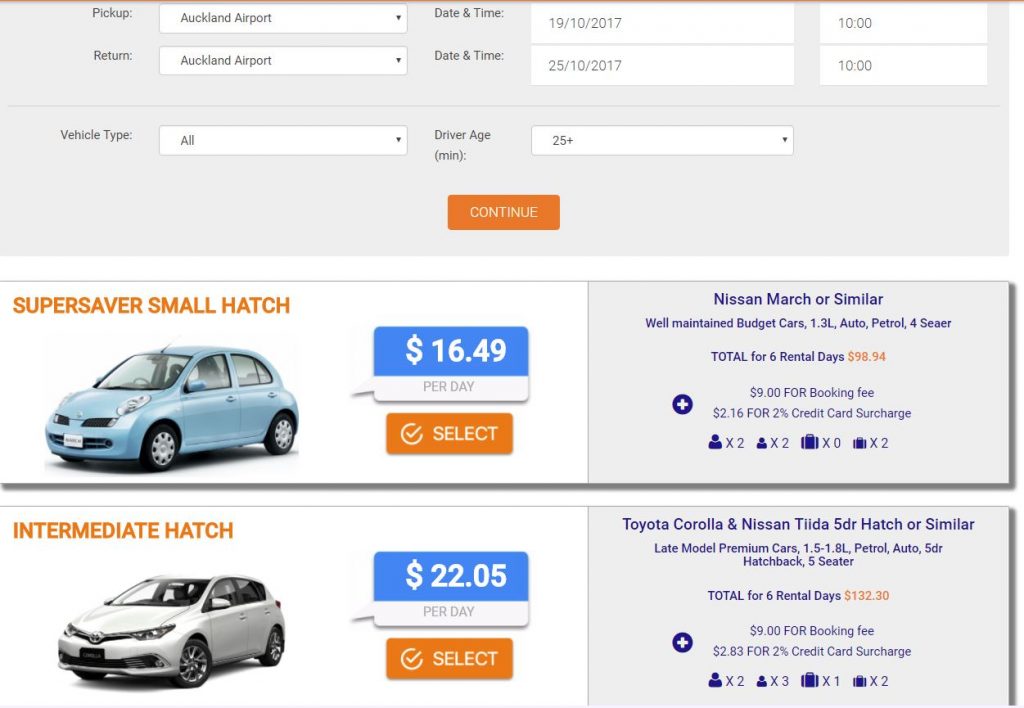On this car rental website, a user has entered their rental criteria, specifying pickup and return locations at Auckland Airport, with dates from October 19, 2017, to October 25, 2017. They have left the vehicle type as any or all, and the driver's age is specified as 25 years old. Upon clicking "Continue," the site displays available car options for the requested dates.

The first available car is a Super Saver Small Hatchback, described as a well-maintained budget vehicle, comparable to a Nissan March. It features a 1.3-liter automatic petrol engine and seats four passengers. The rental cost is $16.49 per day, totaling $98.94 for six days.

The second available option is an Intermediate Hatchback, which may be a Toyota Corolla or Nissan Tilda, both five-door models or similar. This vehicle is priced at $22.05 per day, with a total rental cost of $132.30 for the six-day period.